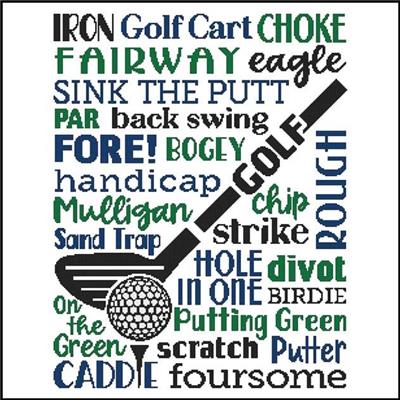This poster features a central image of a black, diagonal golf putter with the word "golf" on it, and a golf ball perched on a tee, which cleverly forms the "I" in the word "caddy." Surrounding the putter and ball are various golfing terms in an array of fonts, including phrases like "iron," "golf cart," "choke," "fairway," "eagle," "sink the putt," "par," "backswing," "bogey," "handicap," "mulligan," "sand trap," "chip," "strike," "hole in one," "divot," "rough," "birdie," "putting green," "scratch," "putter," "foursome," "on the green," and "caddy." The text is featured in a mix of blue, black, and green colors against a white background, with some words aligned in varied orientations and styles, ranging from loopy to blocky lettering.